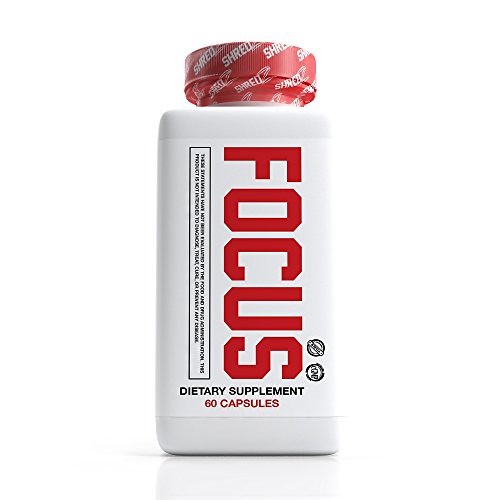This photograph features an unopened bottle of Focus Dietary Supplement, specifically designed to enhance concentration. Encased in a white plastic, square-shaped bottle, it contains 60 capsules and remains securely sealed with the safety shrink-wrap intact on the top. Prominently displayed on the cap is a red seal with bold white lettering spelling out "SHRED," complete with a creatively stylized Z at the end. The label showcases the brand logo, along with other branding elements and detailed product information, set against a stark white background.